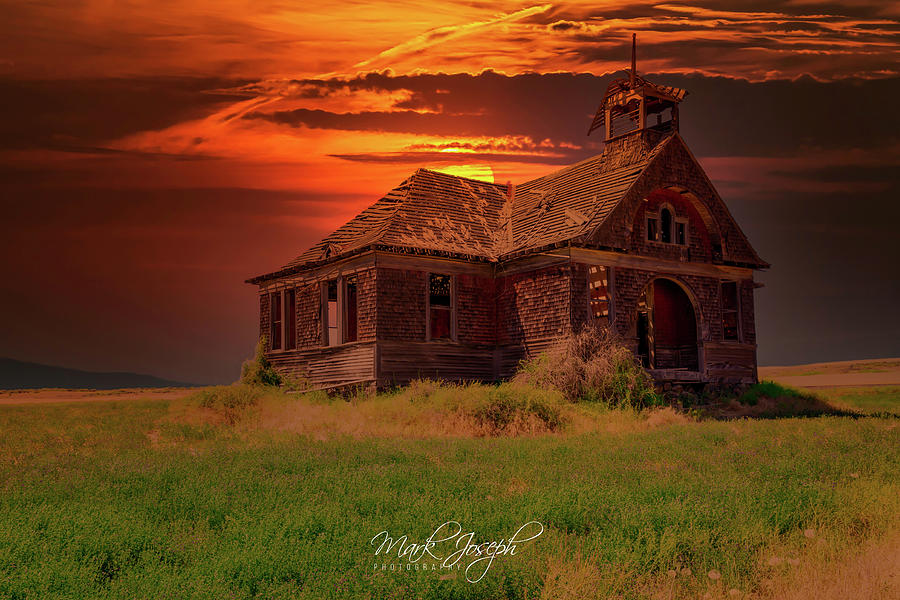In the center of this captivating photograph lies an old, dilapidated house or possibly an old church or school, standing solitary in a small, grassy field. The structure features a roof that is visibly collapsing, with shingles missing and wooden siding falling off. Brick walls interspersed with wooden elements add to its weathered look. The house also includes an archway with a window above it, and a weather vane atop the roof. 

Surrounding the house is a mix of brown and green grass, emphasizing the isolation of this desolate scene. In the far distance, the silhouette of a mountain range is faintly visible. The sky above is breathtaking, with dark gray clouds and vivid tones of orange and yellow, indicating that the sun is setting. This creates a dramatic backdrop for the rugged structure. The prevalent dark colors and the twilight sky contribute to a haunting yet beautiful atmosphere. 

At the very bottom center of the image, the text "Mark Jacob Photography" is clearly written in white. The overall palette includes rich browns for the house, golden hues in the sky, and varying shades of green and brown in the grass, making the scene both somber and strikingly picturesque.